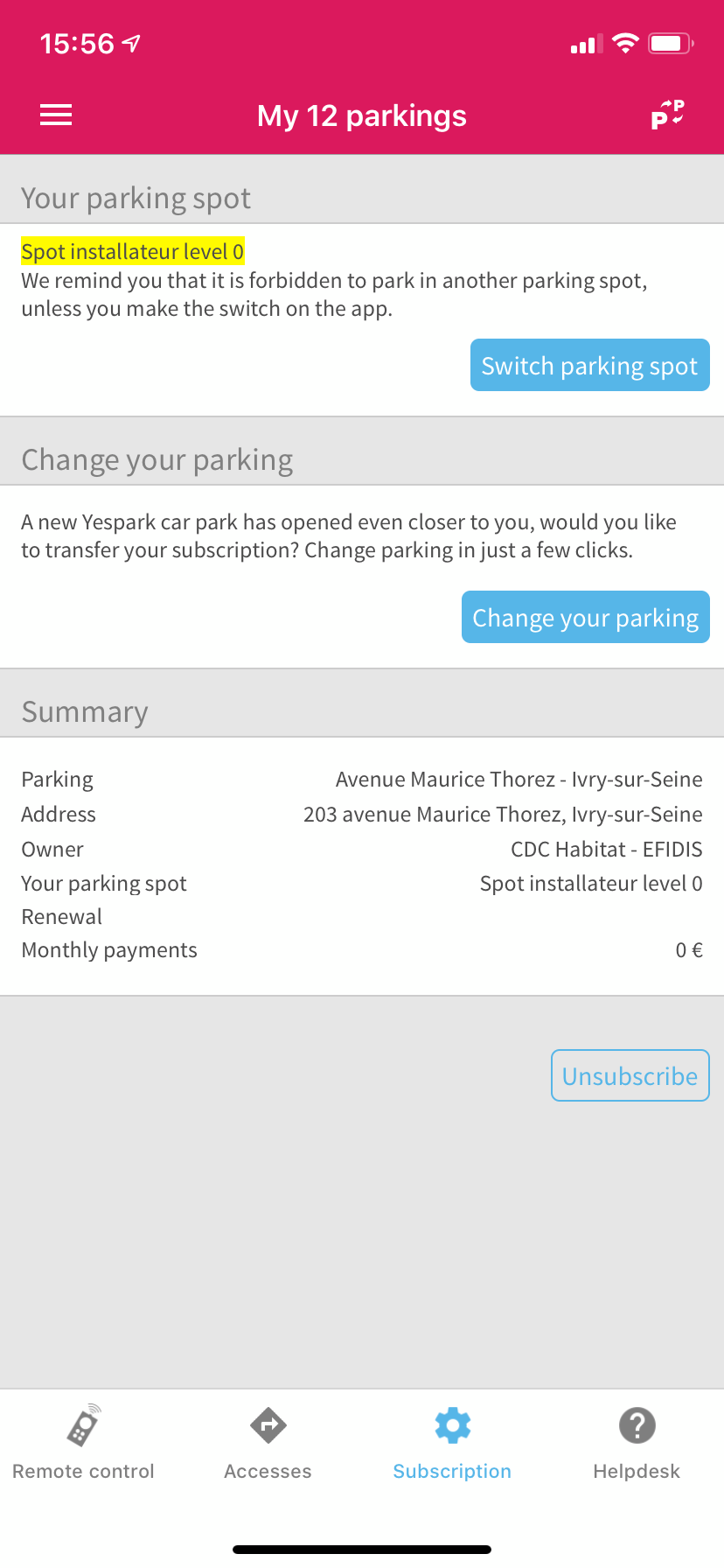**Detailed Image Caption:**

The image depicts a detailed interface for managing parking spot subscriptions. At the top of the interface, the time is displayed as 15:56, indicating the current time. Location services are active, and Wi-Fi is fully connected. A numerical identifier, 123, is visible alongside these indicators. Below this, there is a link represented by a horizontal line.

The text within the interface suggests it is designed for toll parking management, emphasizing that the user's parking spot is on level zero. It reminds users that parking in a different spot is not allowed unless a switch is made.

A notification announces the opening of a new eSpark car park nearby, offering an option to transfer the current subscription. The action to change parking involves a simple process described as occurring in just a few clicks. The summary section includes details like:
- Parking Location: Avenue Maria Torres, Ivory Sur Sain
- Address: 203 Avenue Maria Torres, Ivory Sur Sain
- Owner: CDC Habitat, EFDIS

The user's parking spot is currently selected at level zero, with no renewal details and a monthly payment listed as zero euros.

Towards the bottom right of the interface, there is a large gray square with the option to 'Unsubscribe' in blue text. At the very bottom left, there is a remote control icon for additional functionalities, and another icon for access. The subscription indicator is colored blue, with the selected option displayed as a blue gear. An additional help desk feature is shown with a gray circle encompassing a question mark in the center.

At the very bottom of the image, a black bar is centrally positioned, possibly indicating a navigation or menu bar within the interface.